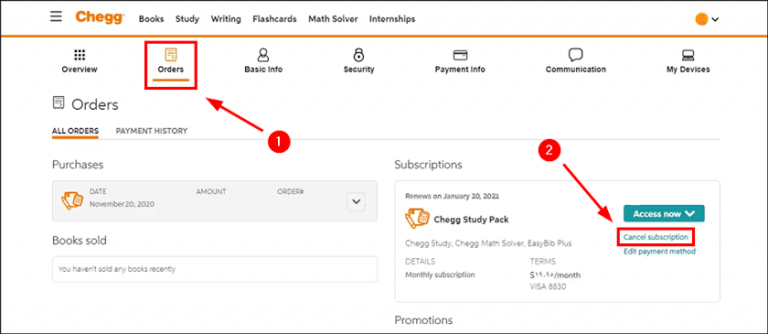Here is a detailed and cleaned-up caption for the described screenshot of the Chegg website:

---

The screenshot captures a user interface of the Chegg website with a clean white background. At the top left corner, there is a three-bar hamburger menu icon. To the right, on the same header with a white background, the Chegg logo is prominently displayed in bold orange font beside the hamburger icon. The header is demarcated from the rest of the page by a long horizontal orange line stretching across the width of the screen.

Next to the Chegg logo, a series of black text dropdown menus are arranged from left to right, labeled: Books, Study, Writing, Flashcards, Math Solver, and Internships. At the top right corner, there's a black downward-facing caret next to an orange circle.

Beneath the primary header, a secondary navigation bar spans from left to right, featuring clickable icons with labels. These include:
1. A grid icon with the label "Overview."
2. A beige piece of paper icon with the label "Orders," underlined in orange.
3. A person icon labeled "Basic Info."
4. A lock icon labeled "Security."
5. A credit card icon labeled "Payment Info."
6. A text box icon labeled "Communication."
7. A computer icon labeled "My Devices."

On the left side, near the middle of the page, the "Orders" section is highlighted with its icon. Below it, the text "All Orders" is underlined in orange next to "Payment History" in light gray. Further below, under the "Purchases" heading, the items that were purchased are displayed. 

In the bottom right section, a rectangular box labeled "Subscriptions" contains details about "Chegg Study Pack," with a corresponding logo. Next to it, a blue turquoise box with white text reads "Access Now," and below that, turquoise text offers options to "Cancel Subscription" and "Edit Payment Method." A red arrow originating from a red circle with the number "2" in white points toward the "Cancel Subscription" option, which is enclosed in a red box.

Additionally, the "Orders" icon at the top left is also highlighted with a red box and a red arrow. This arrow stems from a red circle with the number "1" in white, indicating it as the first point of focus.

---

This caption provides a detailed, step-by-step description of the elements in the screenshot, making it clear and comprehensive.